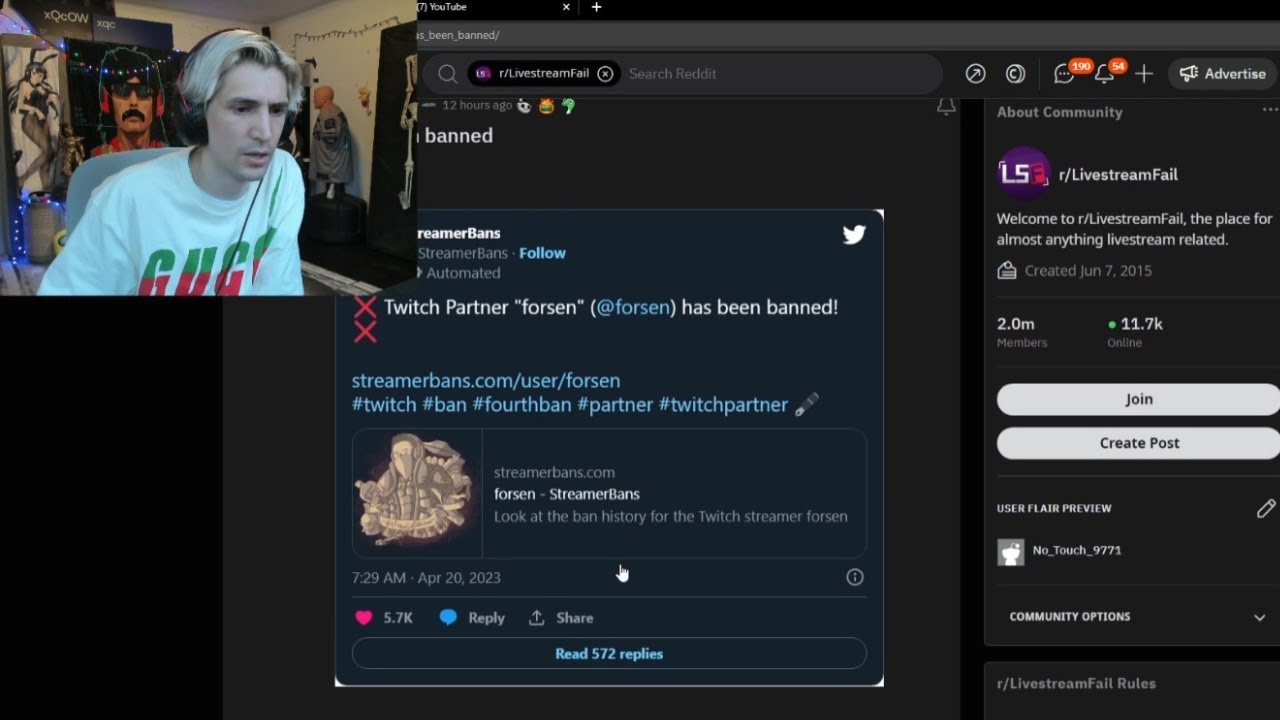In this image, we see a screenshot taken from a live stream. The upper left-hand corner features a face cam of popular streamer XQC, identifiable by the visible letters "XQC" in the background. XQC is wearing a headset and is intently focused on his screen. The main portion of the image displays what XQC is looking at: a Reddit page open to the "r/LivestreamFail" subreddit. The subreddit is described as "the place for almost anything livestream related."

Prominently featured in the Reddit post is an announcement about someone being banned. The post includes a Twitter link from the account "@StreamerBans" with a tweet stating: "Twitch Partner Forsen (@Forsen) has been banned." The tweet provides a URL to the StreamerBans website (streamerbans.com/user/forsen) and includes several hashtags: #Twitch #Ban #FourthBan #Partner #TwitchPartner. The tweet has garnered 5.7K likes and was posted at 7:29 AM on April 20th, 2023.